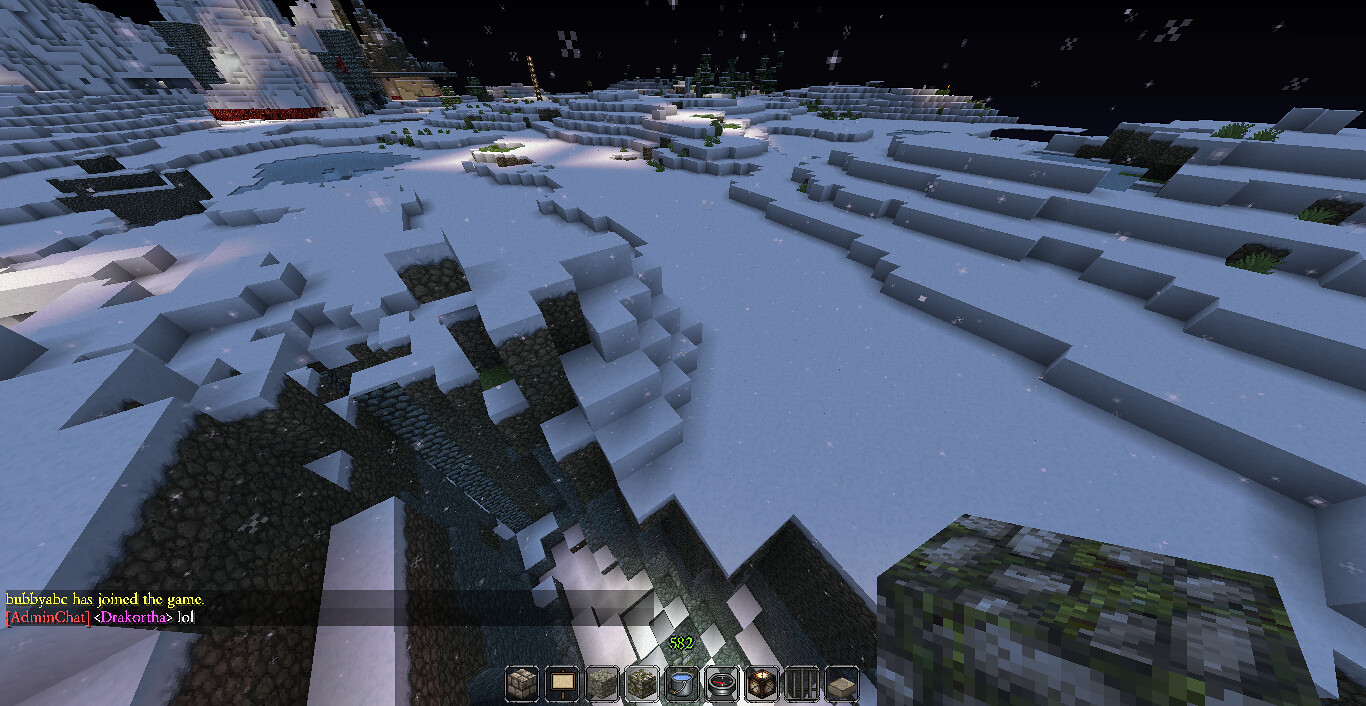In this screenshot from a video game, the setting appears to be a large, snow-covered stadium characterized by numerous dark gray concrete steps that ascend in a grand, circular fashion. The terrain is rugged, with scattered rocks interspersed among the steps, adding to the cold, mountainous ambiance. Towards the background, there are serene, partially snow-dusted trees framing the scene, contributing to the wintry atmosphere. At the bottom of the image, a HUD (Heads-Up Display) features vibrant yellow, red, and purple letters, likely indicating an area where players enter or receive information about the game. The bottom portion of the screen also displays various icons, each representing different aspects or items within the game, essential for guiding the player's actions.